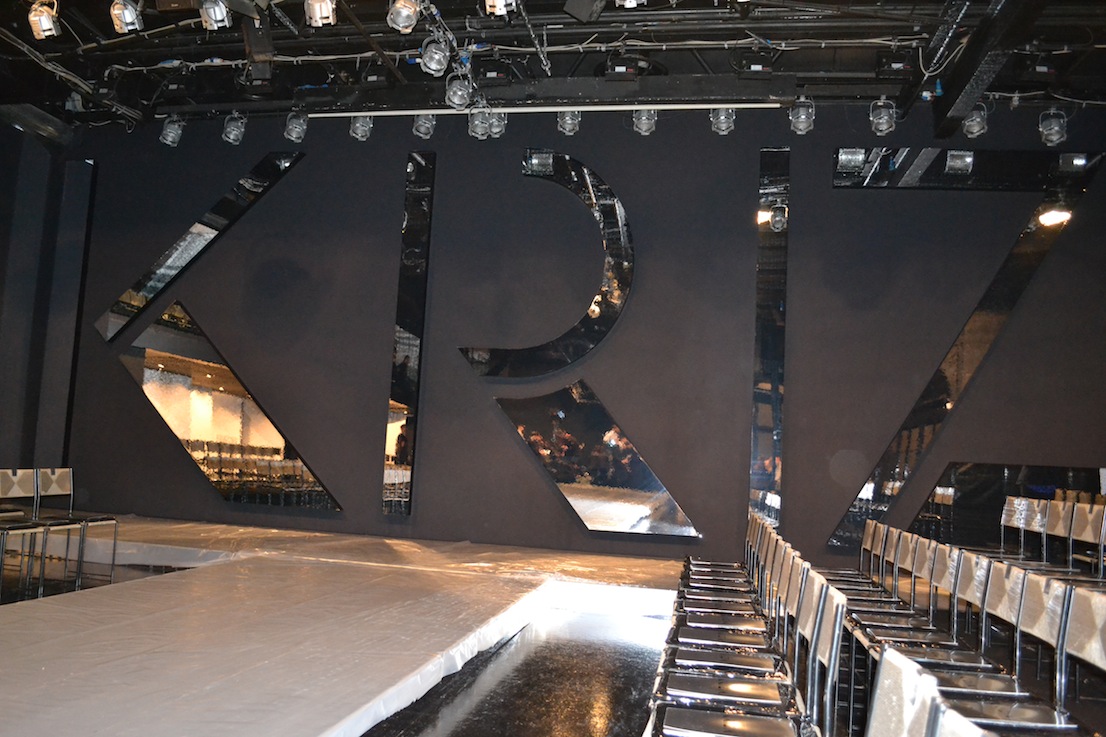The image depicts the interior of a sleek, modern fashion show venue. Dominating the scene is a pristine, white catwalk running parallel between rows of meticulously arranged silver chairs on either side, though the right side is more visible. Above, numerous track lighting fixtures and large studio flash bulbs illuminate the space, reflecting off the mirrored, abstract decorations on the dark gray, almost black, back wall. These mirrored elements, possibly forming the angular and curved letters K-R-I-Z, add an artistic flair to the setting. The ceiling is a network of black beams, contributing to the high-fashion atmosphere. The overall lighting, including lights positioned below the stage, creates a bright, reflective ambiance that captures the modern elegance of the venue.